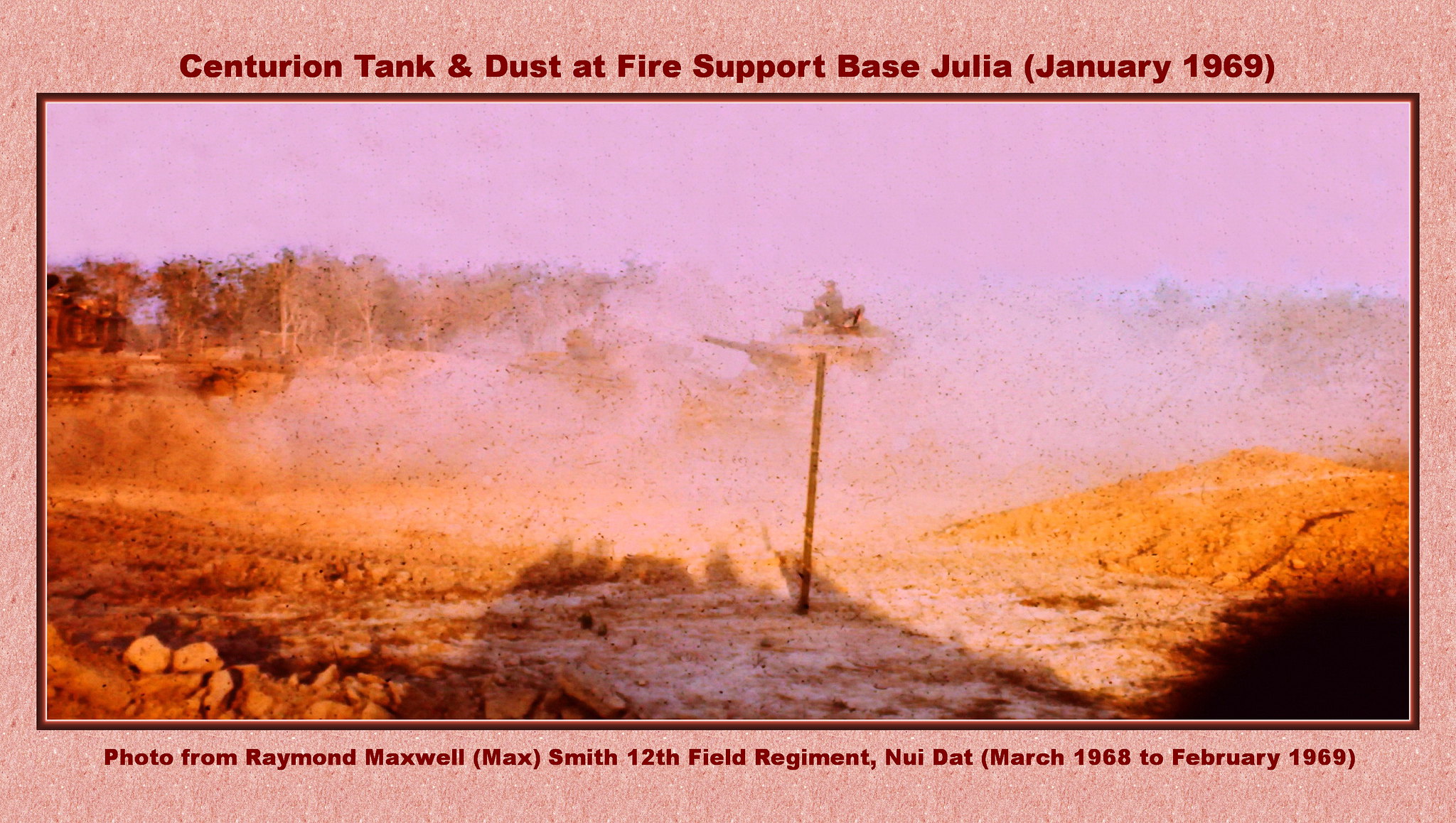The image is a photograph with a peach-colored border featuring maroon text at the top that reads, "Centurion Tank and Dust at Fire Support Base Julia (January 1969)." The photo, credited to Raymond Maxwell "Max" Smith from the 12th Field Regiment, Nui Dat, March 1968 to February 1969, is set against a speckled red and white background. The scene depicts a rugged, earthy terrain in a rusty brown or golden shade, stretching across the entire area. In the background, a tree line is partially visible, shrouded in a pervasive, thick smoke or haze that dominates the middle and right portions of the image. Through this dense cloud, the silhouette of a Centurion tank can be discerned, with a soldier visible atop the hatch. The overall ambiance suggests a moment captured in the midst of action, emphasizing the dust and chaos of the portrayed military scene.